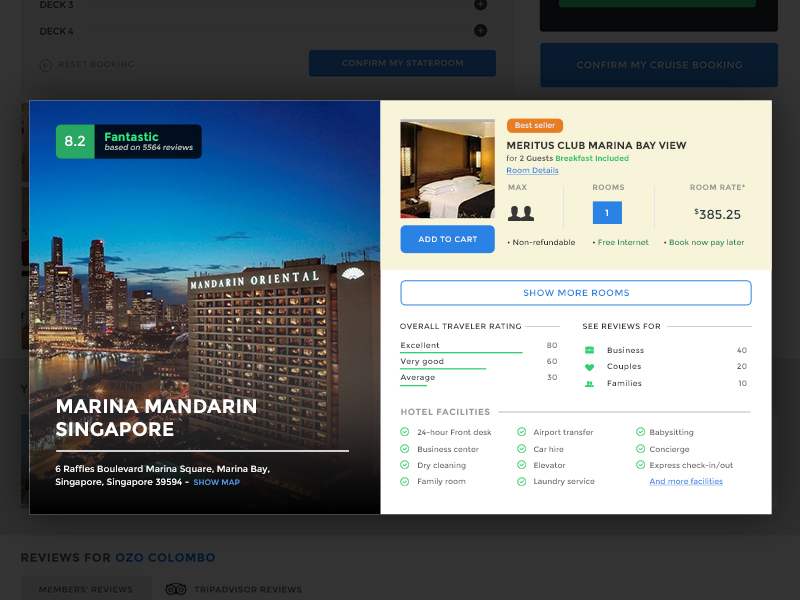The image is a screen capture of a travel booking website interface. The main background is grayed out, over which a prominent white webpage is displayed. This display features various blue and white icons. There are two highlighted options on the gray overlay: one box marked "Confirm my state room" and another marked "Confirm my cruise booking." Towards the bottom, there's a section titled "Reviews for OZO Colombo," including "Member Reviews" and "TripAdvisor Reviews."

Overlaying this background, a detailed pop-up showcases information about "Mandarin Oriental." On one side, there's an image of a grand, ornately designed hotel with illuminated windows, surrounded by lit skyscrapers, under a night sky with clouds, and a body of water and traffic below. The pop-up text reads, "Mandarin Oriental Marina, Singapore, 6 Raffles Boulevard, Marina Square, Marina Bay, Singapore, Singapore, 39594," accompanied by a blue "Show Map" button.

At the top of this pop-up, a ratings box is displayed. It is in white, green, and black, with "8.2 Fantastic" based on several thousand reviews. Adjacent to this is another image in a tan box depicting a hotel room with white bedding. This section includes an orange and white label "Best Seller" for "Meredith's Club Marina Bay View," suitable for two guests with breakfast included. A blue "Room Details" button can be clicked to reveal further details: maximum two people, one room, priced between $385 and $525 per night, a "Book Now Pay Later" option, free internet, and noting that the booking is non-refundable. Below this image, there is a blue and white "Add to Cart" button and another box to "Show More Rooms."

The pop-up also provides an overall traveler rating: excellent (80), very good (60), average (30), including categories such as business (40), couples (20), and families (10). A detailed list of hotel facilities, each marked with green checkmarks, includes a 24-hour front desk, business center, dry cleaning, family room, airport transfer, car hire, elevator, laundry service, babysitting, concierge, and express check-in and out, with an option to view more facilities.